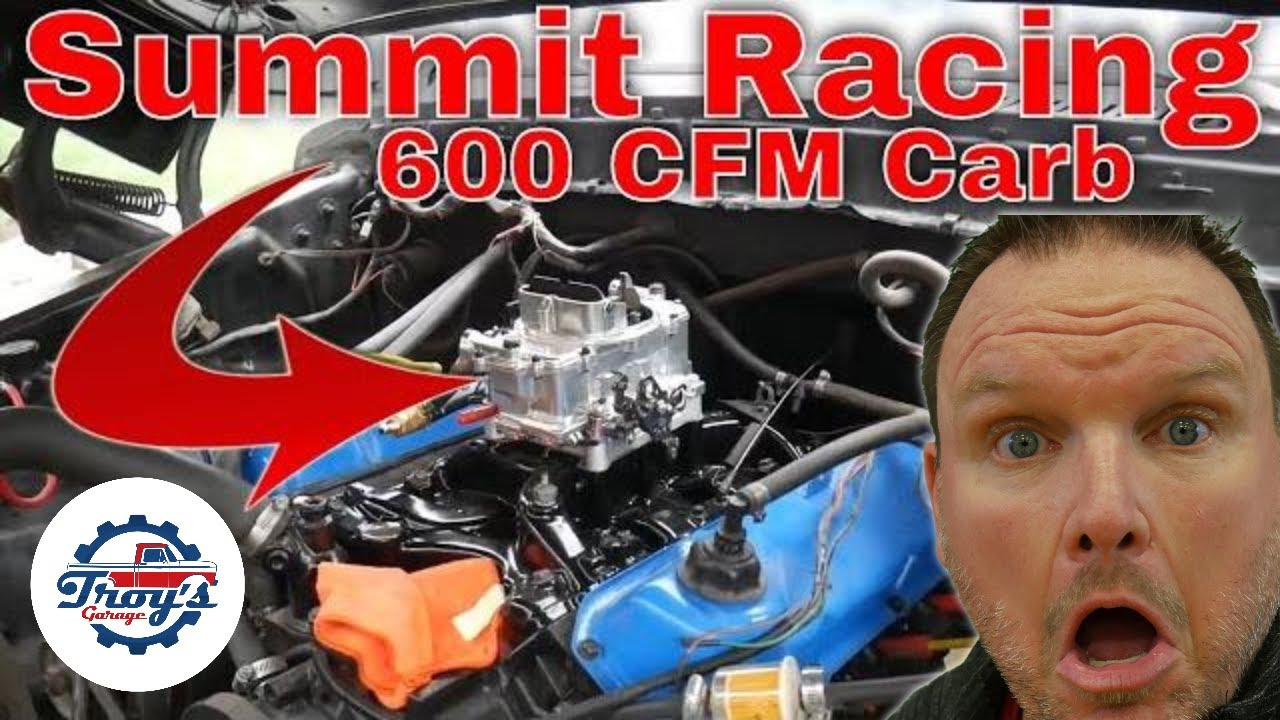The image appears to be a promotional YouTube thumbnail for Summit Racing, showcasing a 600 CFM carburetor. At the top of the image, in bold red text with white outlines, it reads "Summit Racing 600 CFM Carb," accompanied by a large red arrow pointing to the center of the engine. The engine itself is prominently displayed with the hood up, featuring a silver cube-like structure at the top, followed by a black section with visible wires and metal parts, and an orange part of the engine lower down. To the right of the engine, a blue tube-like structure is connected. In the lower left corner, there's a circular logo for "Troy's Garage," depicting a red pickup truck encircled by a gear, with "Troy's" in blue and "Garage" in red. In the lower right corner, a close-up of a middle-aged Caucasian man with blue eyes, short hair, and a receding hairline shows him with an expression of shock, mouth wide open, possibly indicating surprise or excitement at the featured product.